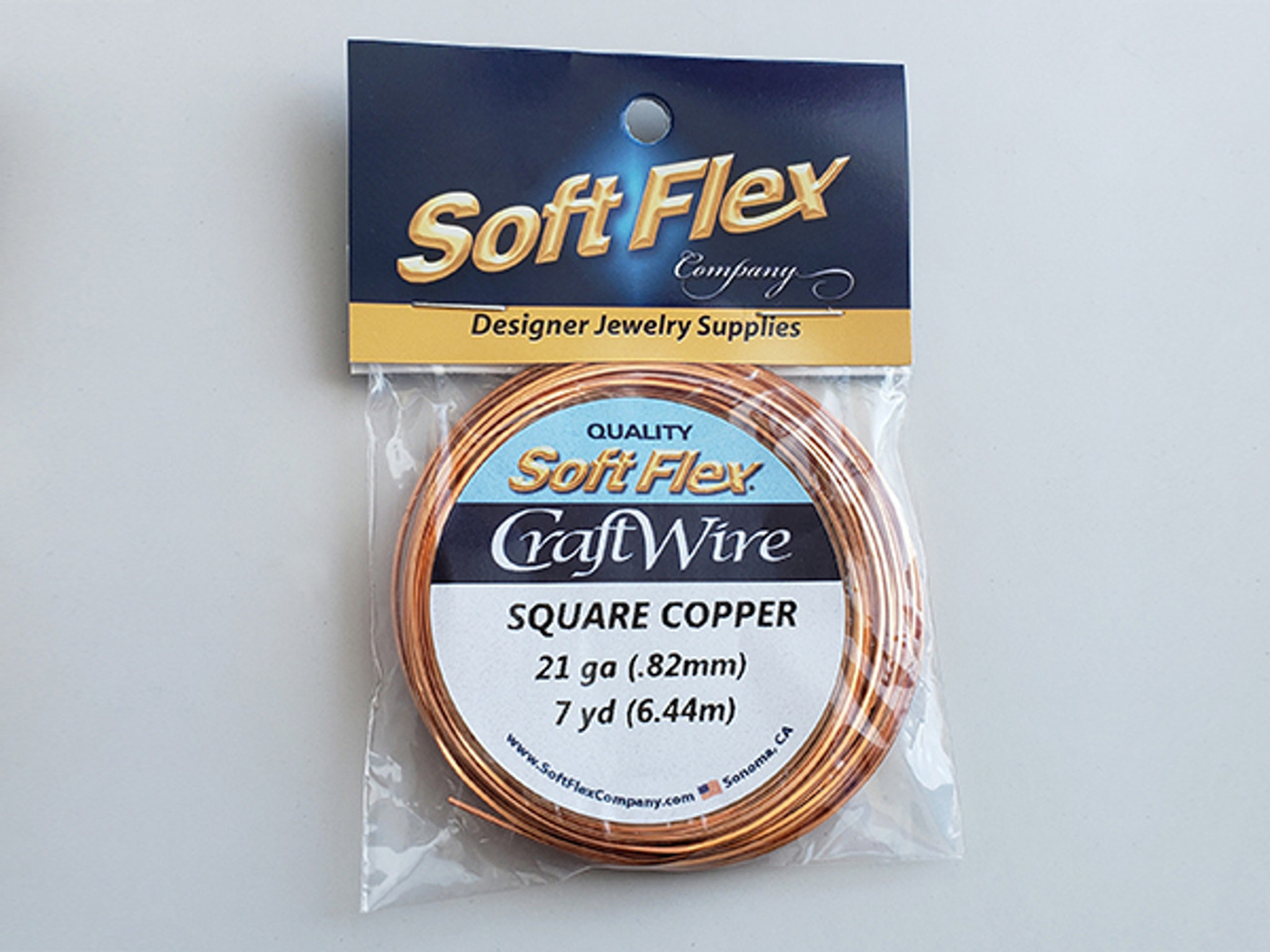This image features the packaging of SoftFlex Company Designer Jewelry Supplies, specifically showcasing their quality craft wire in square copper form. The package contains a 7-yard spool of 21-gauge (0.822 mm) copper wire, neatly wrapped in a circle and enclosed in a clear plastic bag. The top of the bag is sealed with a folded cardboard label stapled through the plastic, designed for hanging in a retail store.

The primary label features a blue background with “SoftFlex” embossed in gold 3D letters, and below, a yellow section with blue text that reads, “Designer Jewelry Supplies.” The spool itself is adorned with a light blue label, which includes various text segments: "Quality" in black, “SoftFlex” in a repeating format, “Craft Wire” in blue script, and finally, “Square Copper 21 Ga, 0.822 mm, 7 yards, 6.44 meters” in black text. Additionally, in small blue letters, the website www.softflexcompany.com is listed, along with an American flag symbol and the location “Sonoma, California.”